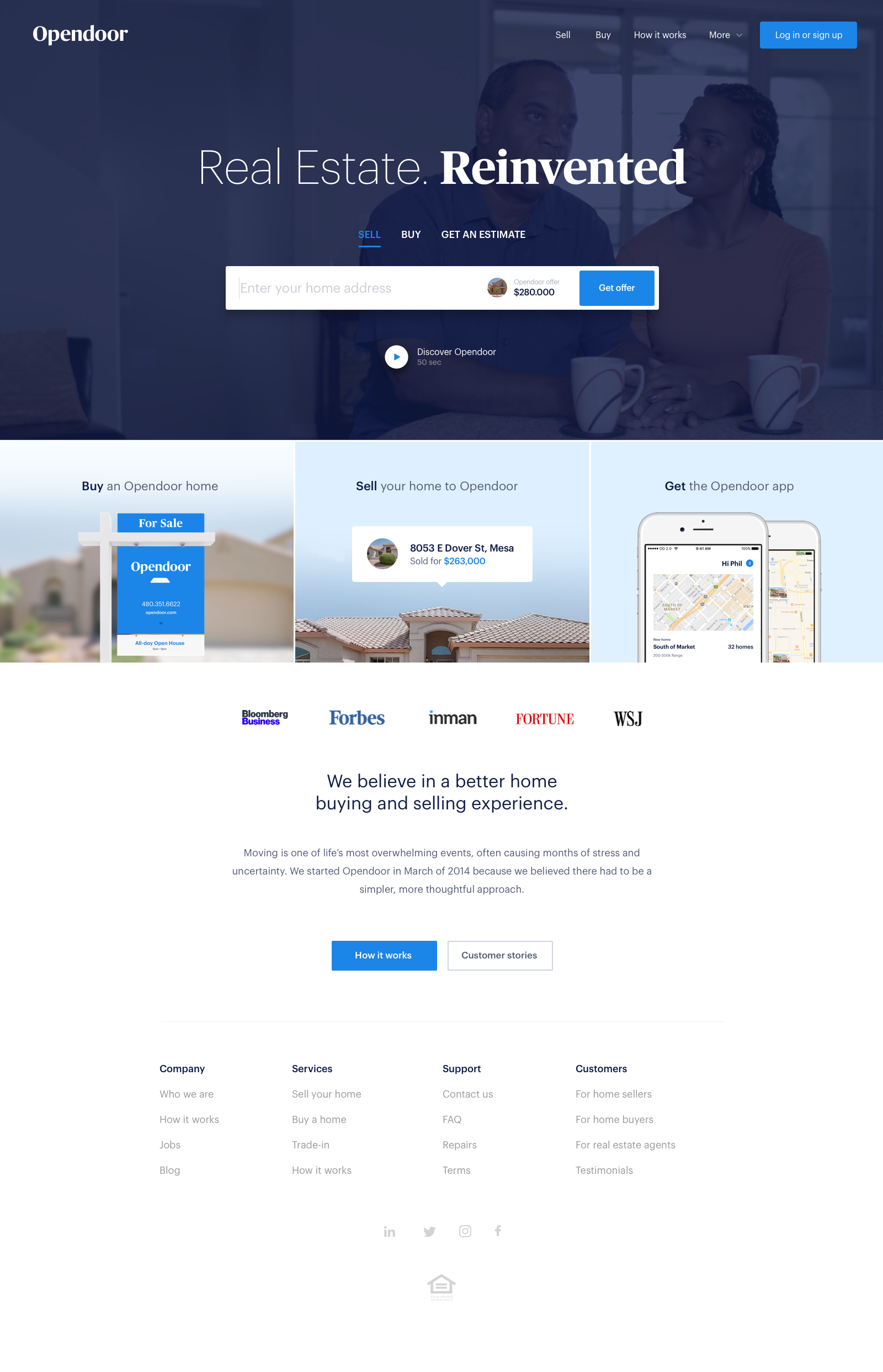The image depicts a real estate website, prominently featuring the company name "Open Door" in small white letters at the top-left corner on a partially transparent overlay. The backdrop consists of a photograph of people, lending a human touch to the digital interface. 

At the top-right corner, navigational tabs labeled "Sell," "Buy," "How It Works," and "More" (with a drop-down option) are neatly arranged. Adjacent to these tabs is a blue button with white text that reads "Log In or Sign Up."

Centrally displayed in large white letters are the words "Real Estate Reinvented." Just below, three options are presented: "Sell" in blue text with an underline, "Buy" in white, and "Get an Estimate" also in white.

Moving further down, there is a rectangular input field framed by a circle icon featuring a house image. Inside the rectangle, the prompt "Enter Your Home Address" is displayed, followed by an estimated offer of "$280,000" from Open Door. A blue-button with white text below this box invites users to "Get Offer."

At the bottom of the page, the layout is divided into three informational blocks: "Buy an Open Door Home," "Sell Your Home to Open Door," and "Get the Open Door App," each providing easily accessible call-to-action sections for users.